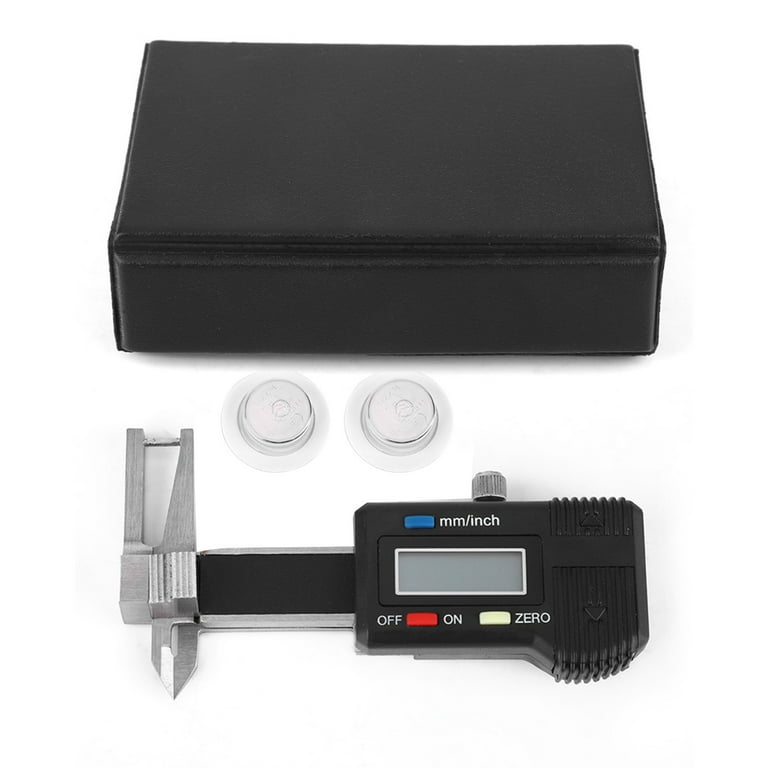This is a detailed stock photo of an electronic caliper set against a white background. The caliper itself is predominantly black and silver, composed of metal with plastic components. The black plastic case is displayed separately at the top of the image. The case features an empty LCD screen and various control buttons, including a blue button labeled "mm/inch" for unit conversion, a red button for powering on and off, and a white button for re-zeroing the display. A silver manual adjustment knob is also visible on the top of the case. Below the case are two small, round discs with holes in the center, serving as attachments or accessories. The caliper, situated to the left of the case, has elongated pointy ends facing downward, indicative of its measuring function. The tool consists of a black plastic body with silver metal strips and a digital sliding scale.